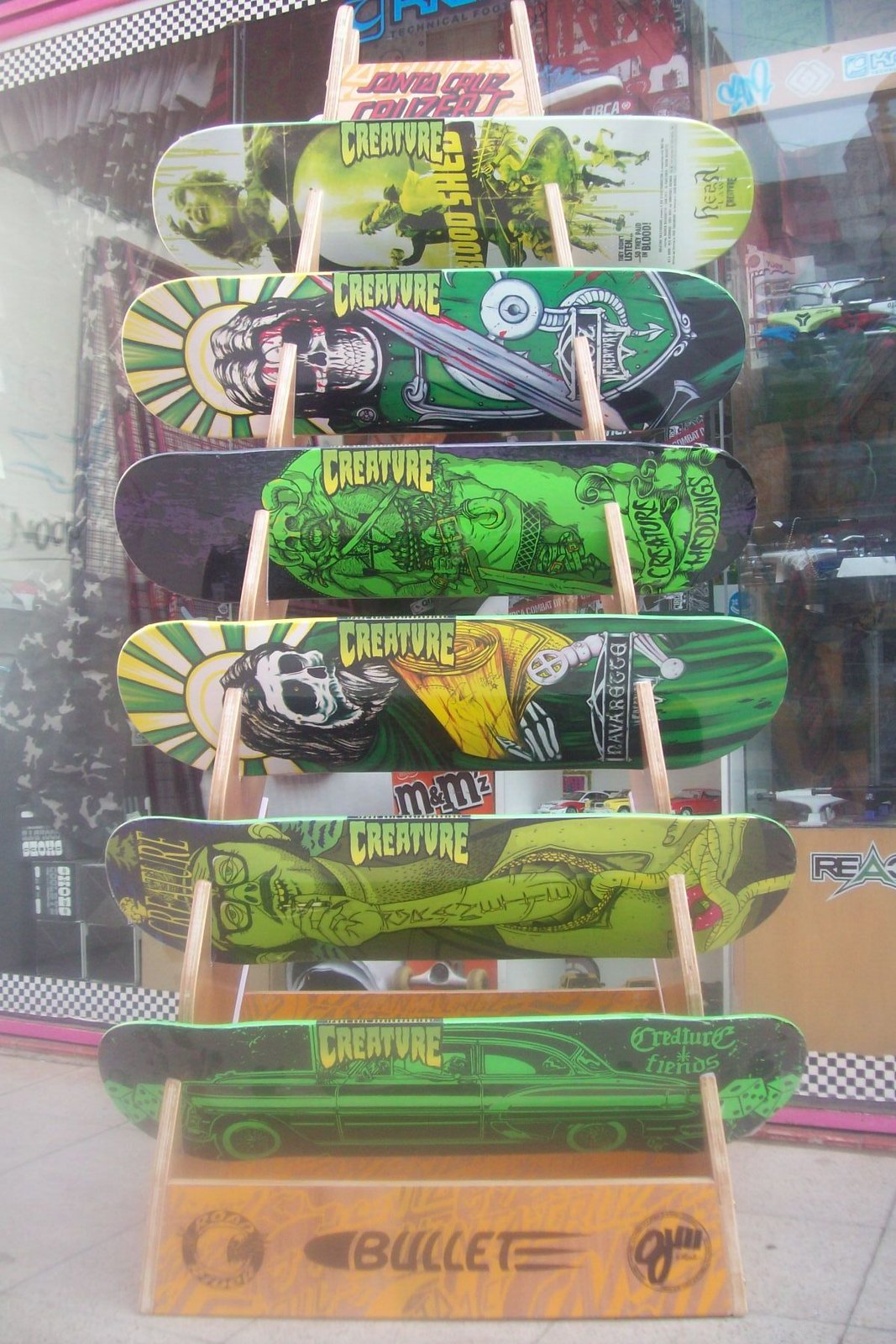In front of a storefront, this image showcases a detailed display of six skateboards without wheels, prominently featuring the brand name "Creature." These skateboards are arranged in a pyramid-shaped wooden rack with cutouts that hold each board at an upward angle, making the intricate designs visible to passersby. Dominated by shades of green with accents of yellow and black, the graphics exude an edgy, punk-like aesthetic. Among the diverse designs, you can spot a tattooed man smoking, shimmering skulls, a fierce-looking car, a woman, an ogre, and figures reminiscent of saints adorned with halo-like sunbeams. Above the display, text reads "Santa Cruz," partially obscured. At the bottom of the rack, "Bullet" is clearly inscribed on a beige wooden surface. The arrangement not only highlights the unique artistry on each board but also enhances the rebellious, vibrant nature of the "Creature" brand.